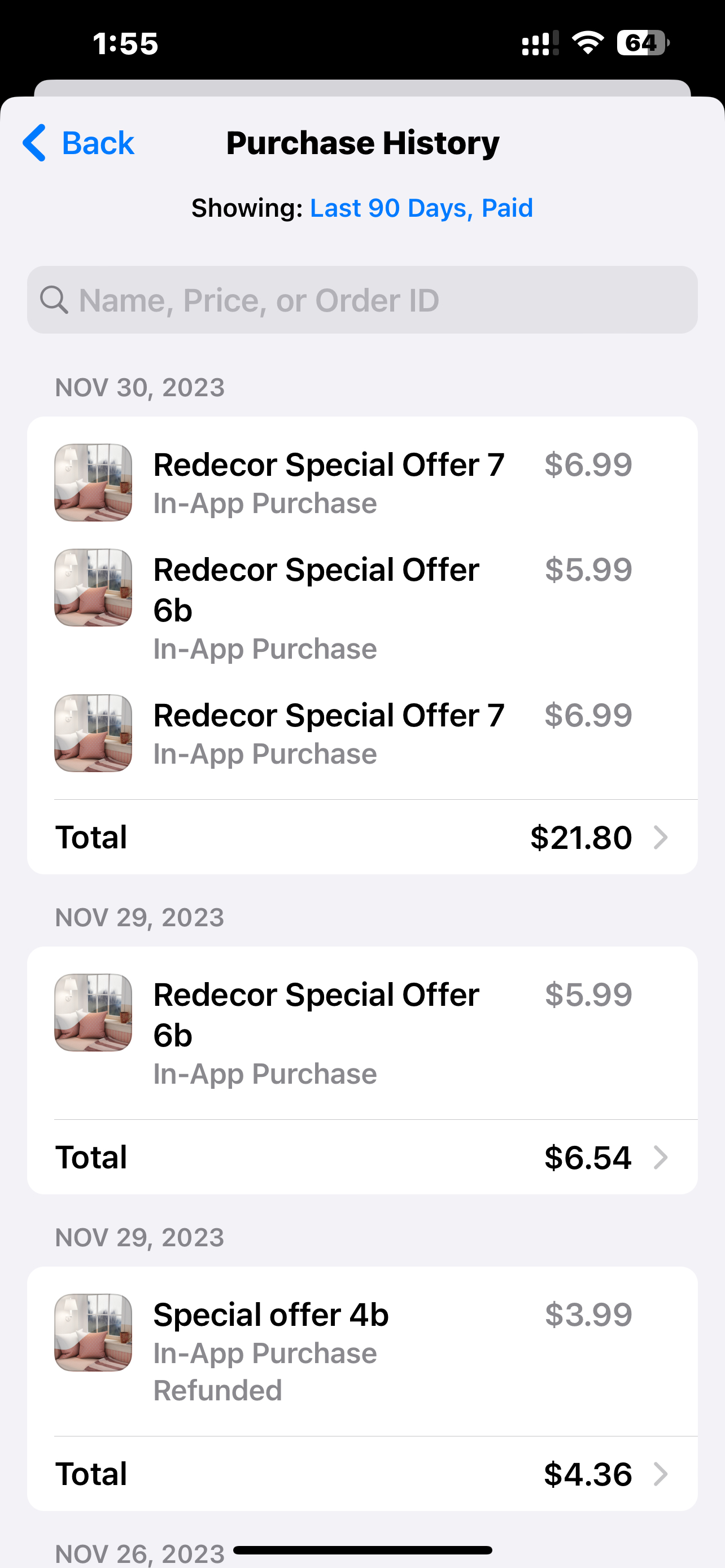This is a screenshot of a smartphone taken on November 26, 2023, at 1:55 PM, displaying the purchase history of an individual for the last 90 days, with a focus on in-app purchases. The user made several transactions for the Reed Decor application. On November 30th, the user purchased three items: two "Reed Decor Special Offer 7" in-app purchases and one "Reed Decor Special Offer 6B" in-app purchase, totaling $21.80. On November 29th, the user bought another "Reed Decor Special Offer 6B" in-app purchase for $5.99, but with taxes, the total was $6.54. Also, on November 29th, a "Special Offer 4B" in-app purchase was refunded; initially priced at $3.99, the user received a refund of $4.36 including tax.